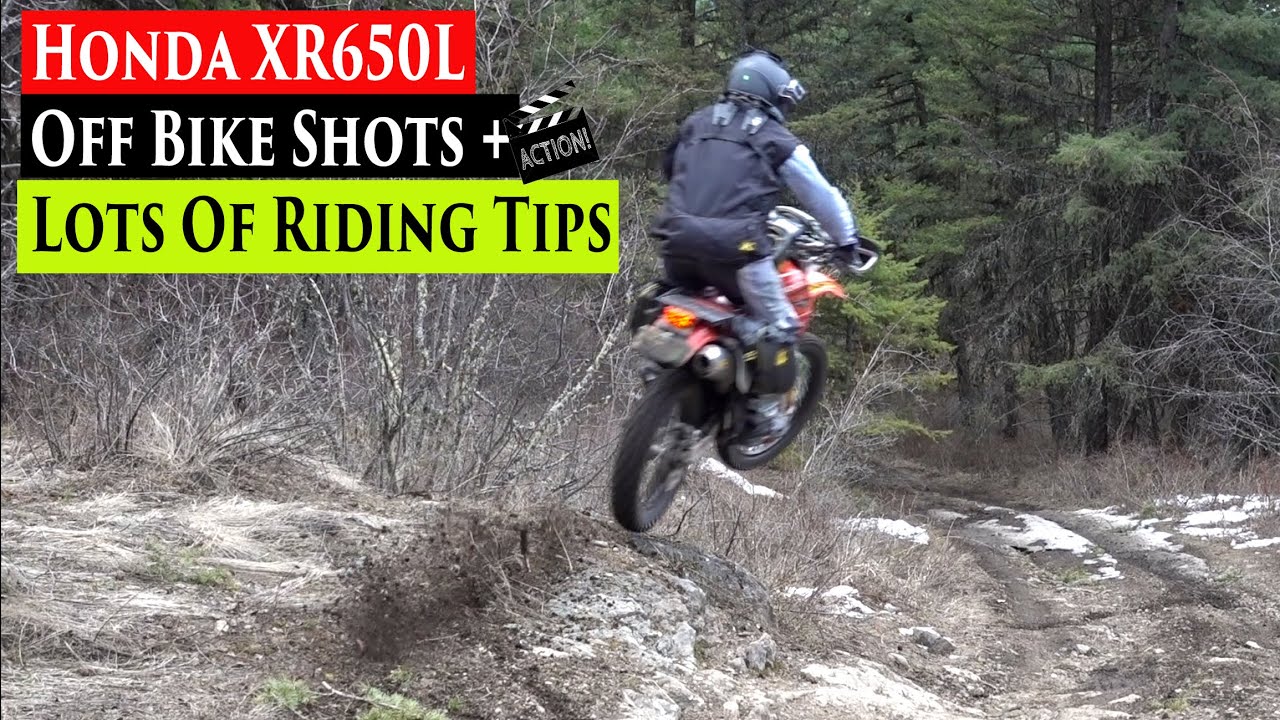This dynamic action shot captures a motorcyclist soaring mid-air on a Honda XR 650L dirt bike, vividly against a rugged, rocky terrain speckled with remnants of snow. The rider, seen from behind, is adorned in a dark jacket with distinct blue sleeves, matching blue jeans, and a blue helmet. His red and black bike propels him over a stony dirt path, with bare-branched trees interspersed with evergreen pines forming a scenic background. The top left corner of the image features a red banner with white text reading "Honda XR650L," followed by a black banner with white text stating "Off-Bike Shots plus Action," complete with a cinematic action clapperboard icon. Below, a green banner with black lettering advertises "Lots of Riding Tips," further situating this thrilling moment within a context of adventure and expertise.